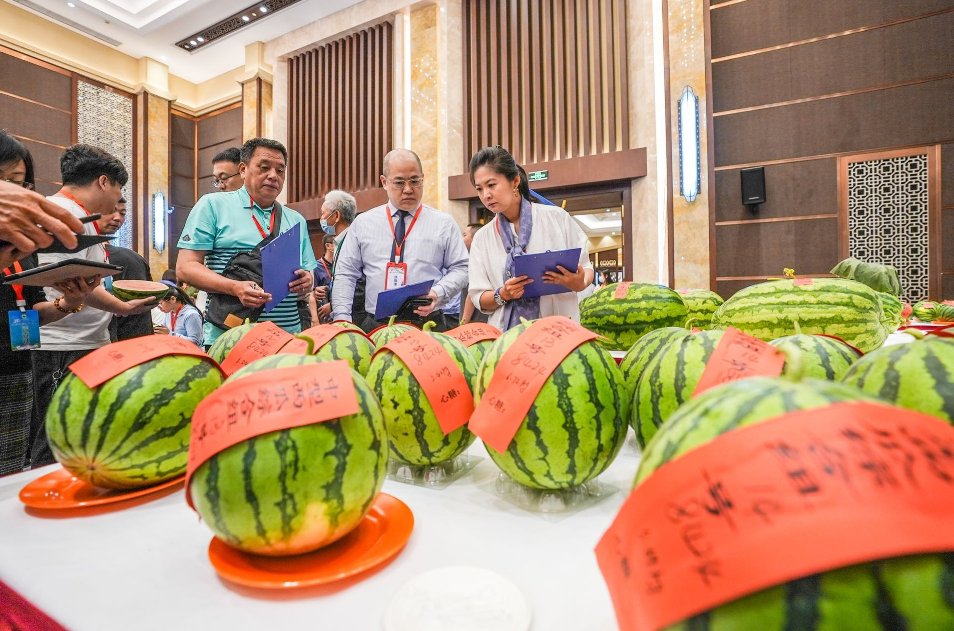This indoor image captures a detailed scene of what appears to be a watermelon judging contest set in a spacious, elegantly designed building with brown and cream tones. At the center, a pristine white table is adorned with various watermelons, many of which are placed on red plates. Each watermelon is marked with a red ribbon featuring Chinese writing, indicative of an international or cultural event. The watermelons themselves are mostly round, with light green skin accented by dark green jagged stripes, though a few oblong ones can be seen in the background. Surrounding the table are three or four judges, dressed in casual attire, who appear to be of Asian descent. They hold purple clipboards and wear tags around their necks, examining the watermelons with serious expressions.